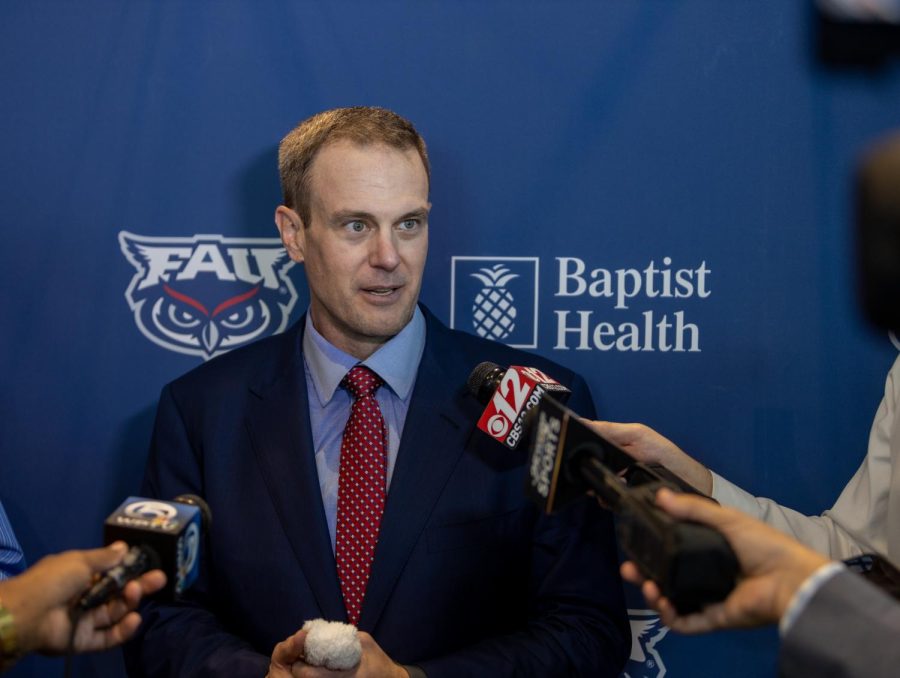The image shows a middle-aged, clean-shaven Caucasian man being interviewed by multiple TV reporters. He has short, grayish-brown hair and is dressed in a dark blue suit, a light blue dress shirt, and a red tie adorned with white and blue patterns. His hands are clasped in front of him, holding something white and fuzzy. The man appears to be speaking, with his mouth slightly open and one eyebrow raised, suggesting he is in the midst of answering questions. Reporters, whose faces are not visible, extend at least three microphones towards him, each marked with different TV station logos. The backdrop features a dark blue cloth with two logos: the owl mascot of Florida Atlantic University (FAU) to his right and the Baptist Health logo, including a square with a pineapple, to his left. This setting, combined with his attire and the context, implies that he is an official or coach at FAU, participating in a press junket.